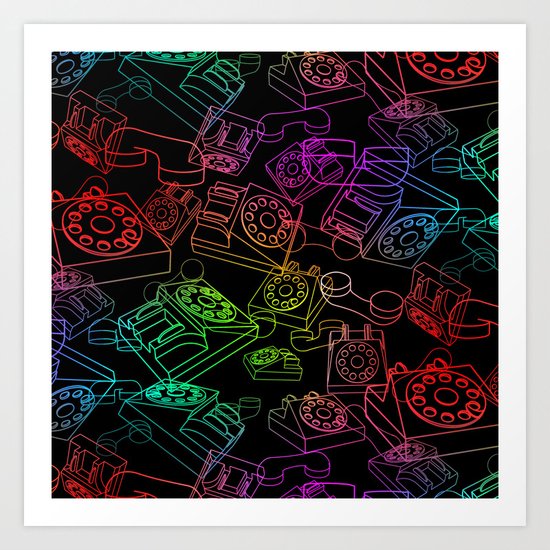The image showcases a striking piece of artwork set against a black background, featuring a vibrant, abstract collage of old-fashioned rotary dial telephones. The central black square is bordered by a double frame—an outer light gray or light blue border and an inner white border, approximately an inch wide. The artwork inside predominantly consists of line drawings of rotary phones, mostly focusing on the base and dials, with only a few handsets scattered among them. These 14 or 15 outlined phones are rendered in a mesmerizing array of neon colors, including red, green, blue, purple, yellow, orange, pink, teal, and peach. The colors often transition within the lines, creating a gradient effect where, for instance, a line may start as red and end as pink. This intricate use of color and light makes the phones appear as if they are glowing in the dark, giving the image an electrifying and almost luminescent quality. The overall composition is a captivating blend of vintage and modern, merging classic telephone shapes with a contemporary, neon-infused aesthetic.